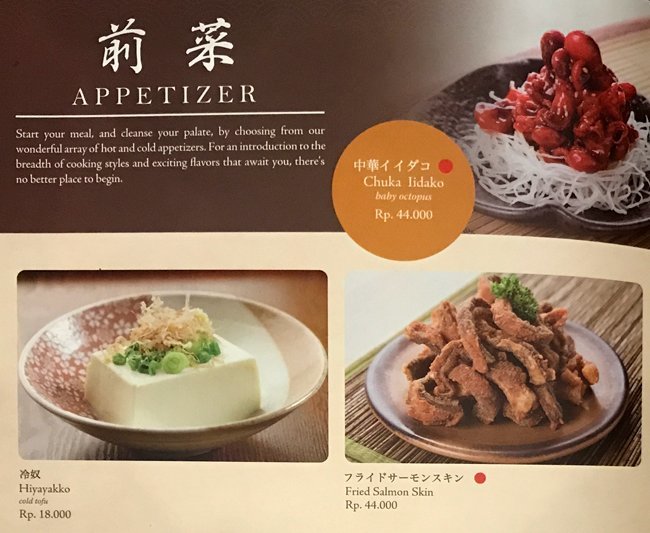The image depicts a page from an Asian restaurant menu, showcasing a selection of appetizers. In the upper left corner, there are two Chinese symbols above the word "appetizer," followed by a detailed description in white text: "Start your meal and cleanse your palate by choosing from our wonderful array of hot and cold appetizers. For an introduction to the breadth of cooking styles and exciting flavors that await you, there's no better place to begin." The menu features three main items:

1. **Chuka Idako (Baby Octopus)**: Displayed in the middle of the image, this dish consists of red, glazed baby octopus over a bed of thin white noodles, priced at RP 44.00.

2. **Fried Salmon Skin**: Situated to the right, on a round brown plate, this item includes crispy fried salmon skins garnished with green leafy vegetables, also priced at RP 44.00.

3. **Haiya Yako (Cold Tofu)**: Located at the bottom left, this dish is presented in a white and brown bowl, featuring a square piece of cold tofu topped with green vegetables and light brown noodles, available for RP 18.00.

The menu text alternates between Chinese and English, and each item is accompanied by a corresponding image and description, emphasizing the diverse and exciting flavors of the appetizers offered.